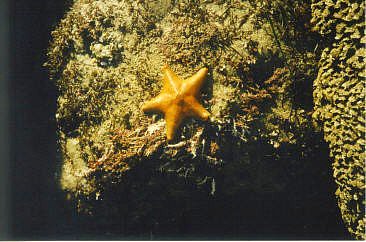This photograph appears to capture a vibrant underwater scene, centered around a striking starfish. The yellow-orange starfish, characterized by its short, thick head prong, is prominently displayed on a rock. This rock, possibly part of a vertically aligned reef or coral wall, is covered in green, moss-like aquatic plant life. The texture of the rock varies, especially on the right side where it extends into a darker, scaly-like formation. The background and left side of the image fade into a pitch-black abyss, accentuating the bright illumination focused on the starfish and its immediate surroundings. There are no other visible plants or animals in the photograph, drawing all attention to the starfish that anchors the scene.